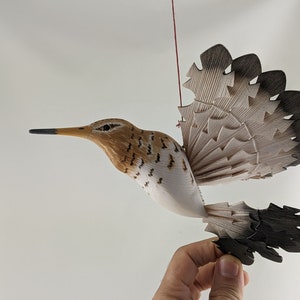This small, square photograph appears to have been taken indoors against a white wall with some shadows. The focal point of the image is a detailed craft representation of a hummingbird, intricately designed and likely carved out of wood. The bird's long beak is black at the tip and transitions to a deep yellow-mustard shade near the head. The body is predominantly brown with a gradient that fades to white on the underside, adorned with a pattern of short dark brown lines. The wings and tail feathers are prominently featured, each displaying a design that starts white and transitions to black at the tips. These feathers are arranged in a way that creates the illusion of natural bird wings and tail. The hummingbird is suspended from a red string, which appears to hang from the ceiling. A hand, slightly darker than Caucasian, is visible in the image, holding the bird by its tail feathers, as if inspecting the craftsmanship. The bird's positioning, combined with the red string and the hand holding it, draws immediate attention to its intricate details and artistic design.